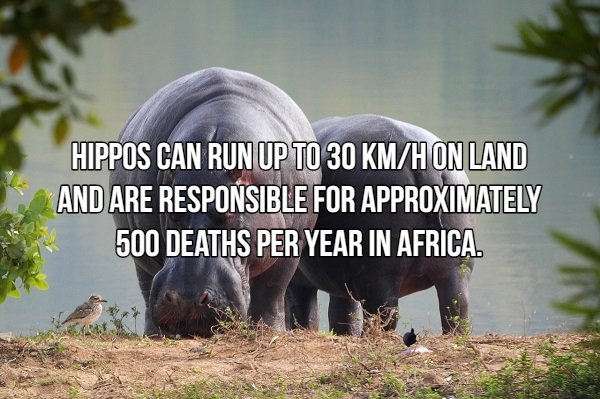In the photograph, two large hippopotamuses stand prominently at the center, each facing a different direction— one towards the viewer and the other away. The hippos, with a shiny, almost purplish-black skin tone, appear to be standing on a riverbank covered with brown, dried grass. Their legs are clearly visible, and one hippo is seen bending down, seemingly eating something from the ground. Adjacent to them, on the left, is a small bird, possibly a swallow, searching for food. The backdrop reveals a still, large body of water, likely a river or lake, extending into the horizon, with a bluish to grayish sky above. Trees frame the scene, with some foliage appearing blurred in the foreground, giving the impression of peering through bushes. The surroundings are distinctly outdoors in the African wilderness, where human presence is rare. Superimposed text in white with a black outline, centrally placed, reads: "Hippos can run up to 30 kilometers an hour on land and are responsible for approximately 500 deaths per year in Africa." The color palette of the image includes browns, greens, grays, whites, oranges, and touches of black, all contributing to the naturalistic vibe of the setting.